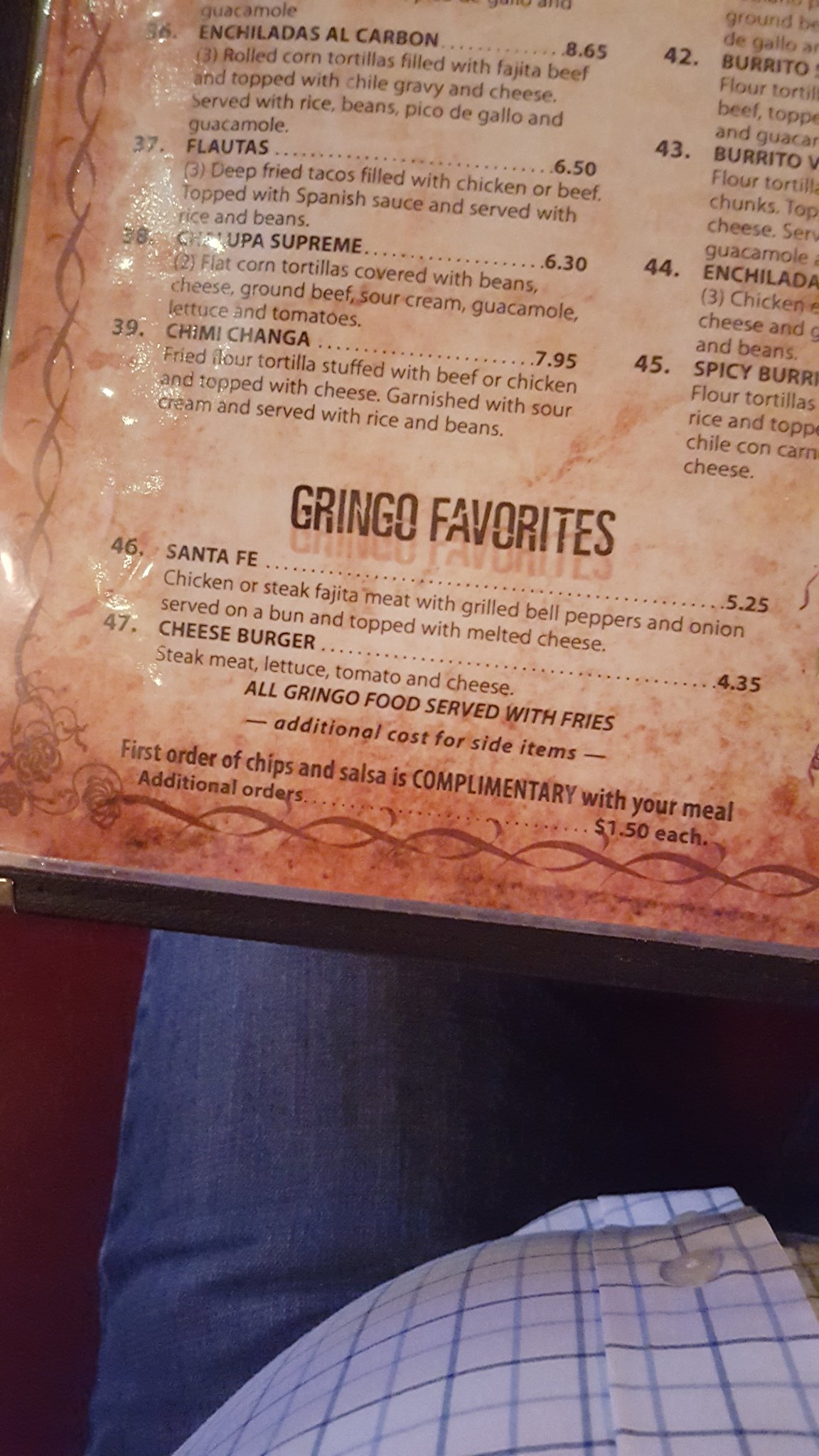This photo captures a detailed view of a restaurant menu, with part of a diner's attire visible in the frame. The person, dressed in a white button-down shirt with blue checkered patterns and blue jeans, is partially visible — displaying their midsection and one leg, likely the left one.

The menu, placed on a table, clearly indicates this is a Mexican restaurant. A selection of dishes is listed, including:

- Enchiladas al Carbón: $8.65
- Flautas: $6.50
- Chalupa Supreme: $6.30
- Chimichanga: $7.95

Interestingly, the menu also features a section labeled "Gringo Favorites." Under this category, the offerings include:

- Cenafé: $5.25 (consisting of chicken or steak fajita meat with grilled bell peppers and onions, served on a bun and topped with melted cheese)
- Cheeseburger: $4.35 (made with steak meat, lettuce, tomato, and cheese)

Additionally, it notes that all "Gringo food" comes with fries, with an extra charge for additional side items. The menu also mentions that the first order of chips and salsa is complimentary, with subsequent orders priced at $1.50 each. The detailed pricing and dish descriptions reflect a thoughtful presentation of the restaurant's offerings.